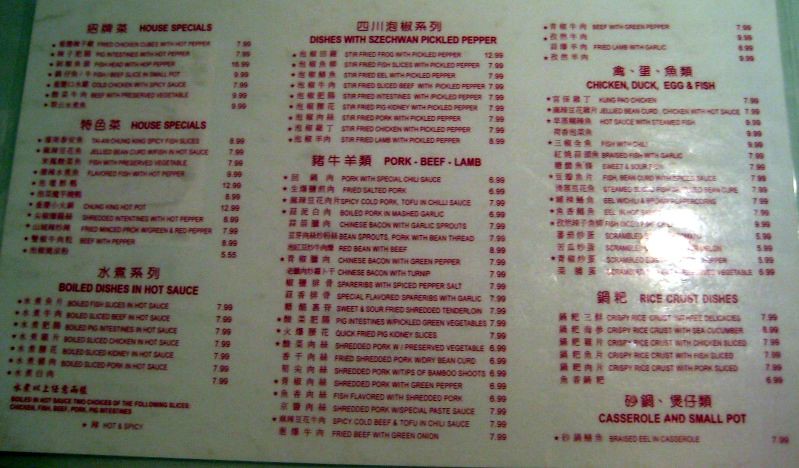On a light blue background, there is a restaurant menu encased in shiny plastic, which reflects a lot of light, giving it a glossy finish. The menu is printed in red letters and is divided into multiple sections. The first section lists the house specials, followed by another section of house specials. Next, there is a category for boiled dishes in hot sauce, with prices neatly lined up alongside the food items. The center section features dishes with Szechwan and pickled pepper, alongside a lengthy list of pork, beef, and lamb options. The third section highlights around four items before moving on to categories for chicken, duck, egg, and fish dishes. There are separate sections for rice crust dishes and casserole and small pot items. Each dish is accompanied by an explanation and is reasonably priced, with many items costing around six to seven dollars.